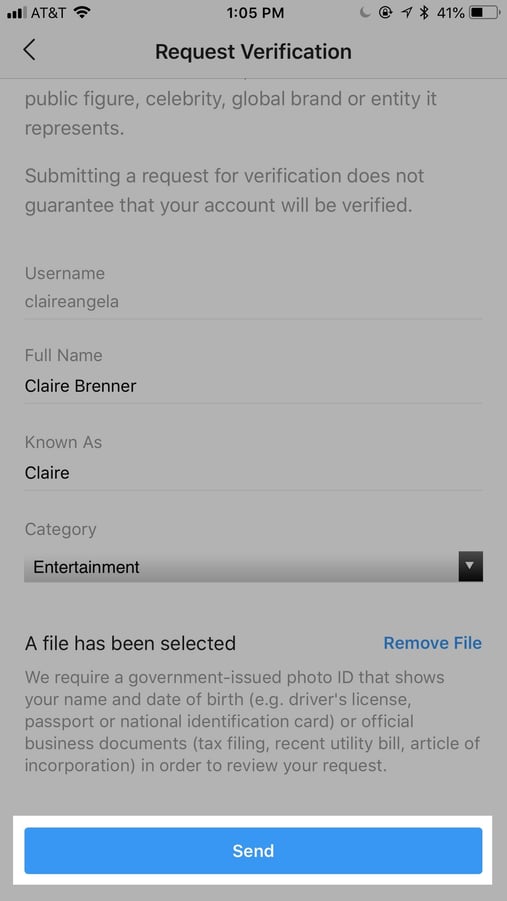The image is a screenshot from a mobile device, likely an iPhone. At the top of the screen, the device displays a 41% battery life, AT&T as the carrier with 4 out of 5 bars of signal strength, and the time is 1:05 PM. 

The majority of the screenshot appears darkened, as if the screen brightness is turned down to approximately 15%. Despite this, you can discern a white background with text in the darkened areas. The focus of the screenshot is a long, rectangular blue button at the bottom of the screen that is illuminated more brightly than the rest of the page. This button features the word "Send" in white text.

In the darker section of the screenshot, there is text indicating the section might be within settings or a similar interface. The text reads, "Request verification," followed by a disclaimer below it: "Submitting a request for verification does not guarantee that your account will be verified." This suggests that the app could be Twitter, as the blue color is consistent with Twitter's branding. The username "ClaireAngelo" and full name "Claire Brenner" are displayed, pointing to the specific user’s account.